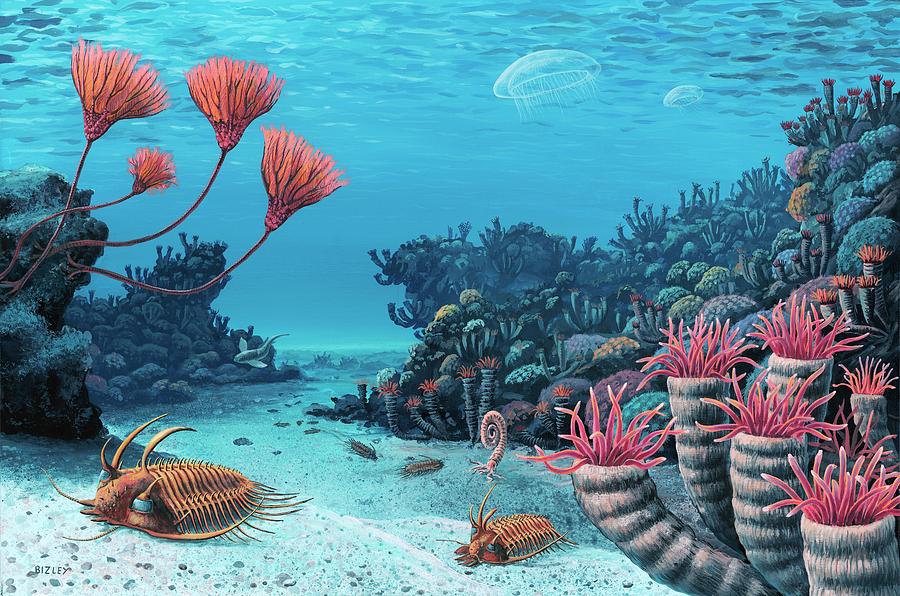The image depicts an animated underwater scene brimming with vibrant marine life. At the top center, a few translucent jellyfish with white hues float gracefully. In the upper left corner, a cluster of underwater plants with long vines rise to culminate in orange-tinted flowers. Below these plants, scattered rocks rest on the sandy ocean floor, which spans the middle and bottom areas of the image. On the left side of the sand floor, a brown, hard-shelled creature, possibly a horseshoe crab, slowly traverses the terrain. The lower right corner showcases tubular pink sea anemones or coral structures, adding to the colorful diversity of the scene.

In the middle of the frame, a coral forest rich in hues of green, orange, purple, and pink stretches towards the backdrop, enhancing the complexity and beauty of the underwater environment. The entire scene is set against a backdrop of blue water, which shimmers with light, capturing the movement and sparkle of the sea.